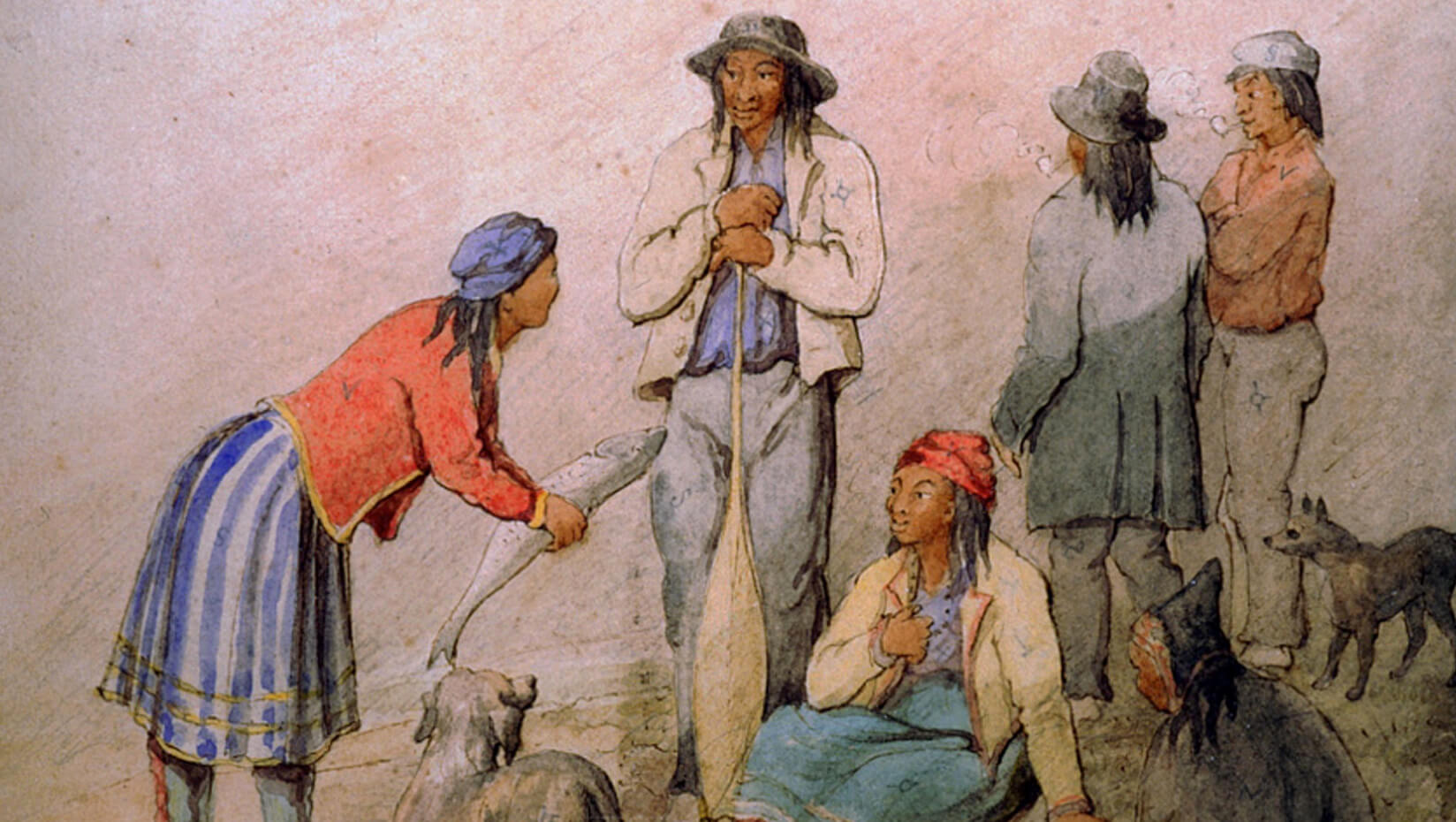This detailed watercolor painting captures an engaging scene of farming activity featuring a group of five people—both men and women—who are dressed in old-time attire. The group consists of four individuals who are standing and one woman seated on the ground. The men are dressed in long-sleeved jackets and grayish pants, with one notable man in the background wearing a white hat. Another man is seen resting his hands on a shovel-like tool. 

Among the women, one is seated on the ground in a yellow jacket and blue overalls, with a red fabric wrapped around her head. Adjacent to her is another woman wearing a red jacket and a blue and white striped skirt, bent over and holding a silver fish, which catches the attention of a blonde dog beside her. The other women are also intricately attired, with one in a black jacket and gray pants, and another in an orange shirt and gray pants, both wearing various hats. These women are engaged in what appears to be a conversation. 

The scene is completed with several animals dispersed throughout, including a black dog looking up at the fish and another dark dog in the background. The detailed attire, tools, and presence of the animals create a vivid depiction of an old-time, rural farming setting, encapsulating the communal effort of gathering food.